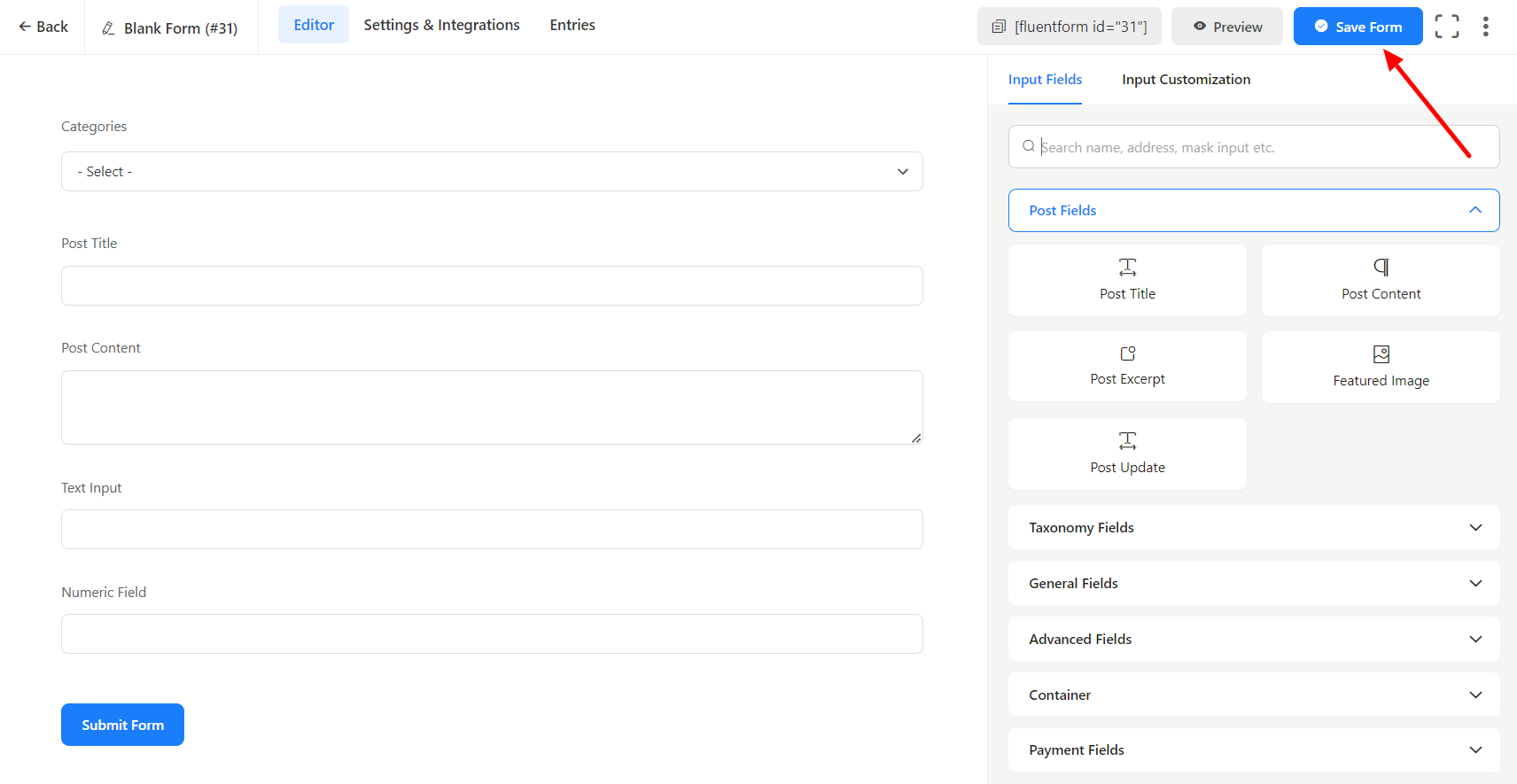**Detailed Caption:**

This screenshot displays the user interface of a computer application page. The top-left corner features a navigation row with several options. Starting from the left, there's a black leftward arrow accompanied by the label "Back," followed by "Blank Form" noted as "(31)." Next to this is a light blue rectangular button labeled "Editor," followed by "Settings and Integrations," and finally "Entries."

Beneath this navigation row, there are five main headings, each associated with a corresponding input area. The first heading, "Category," includes a long gray drop-down bar labeled "Select." The second heading, "Post Title," provides a long gray text box for input. The third heading, "Post Content," features a larger text box equipped with adjustable size bars in the bottom-right corner, allowing the user to resize the input area.

Following that, "Text Input" has an input bar and an additional box below it. "Numeric Field" similarly includes an input box beneath its title. At the bottom of these input sections is a blue rectangular button labeled "Submit Form."

To the right, occupying one-third of the page from the top down, the notation "[fluent_form id="31"]" appears within a gray bar. Directly below this, there's another gray bar labeled "Preview" and a blue bar labeled "Save Form," which is emphasized by a red arrow pointing to it. Adjacent to this are an open square and three vertical dots.

Further down, two categories are displayed: "Input Fields," which is highlighted in blue and underlined, and "Input Customization" in black text. Below these categories is a boxed-off section with a search bar labeled "Search name, address, mask input, etc."

The next element, "Post Fields," is highlighted in blue with a drop-down menu, under which five selectable boxes are listed: "Post Title," "Post Content," "Post Excerpt," "Feature Image," and "Post Update." Additional categories include "Taxonomy Fields," "General Fields," "Advanced Fields," "Container," and "Payment Fields," each accompanied by a drop-down menu.

This thoroughly structured interface appears to facilitate the creation and customization of forms, offering multiple categories and input types for user interaction.